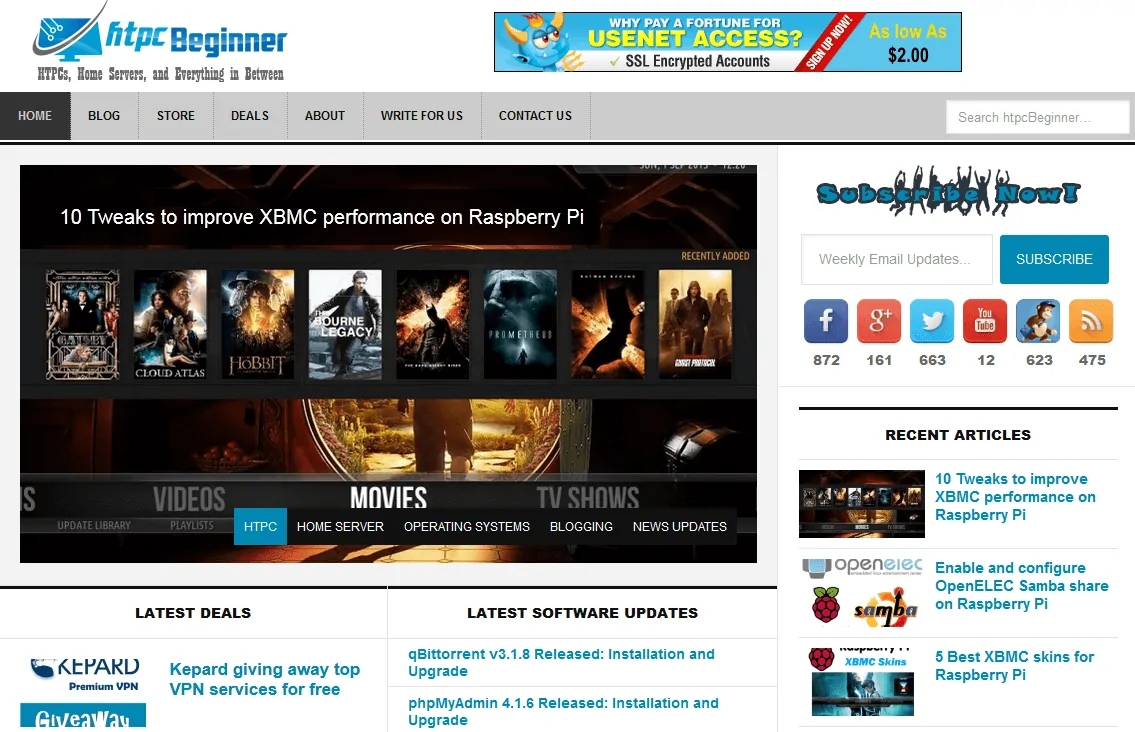This image features the homepage of HTPC Beginner. The central logo prominently displays a computer monitor with a distinctive black swoosh running diagonally from the bottom left to the top right. Accompanying the logo is the tagline: "HTPC, Home Servers, and Everything In Between." 

The top navigation bar, organized from left to right, includes the following tabs: Home (the current page), Blog, Store, Deals, About, Write for us, and Contact us. Positioned at the far right of this bar is a search box labeled "Search HTPC Beginner."

Below the navigation bar is a prominent advertisement highlighting "10 Tweaks to Improve XBMC Performance on Raspberry Pi." Adjacent to this ad are several movie posters and Blu-ray covers, including titles such as "Cloud Atlas," "The Hobbit," "The Bourne Legacy," and "Prometheus." Additionally, there are three more partially obscured titles, one being a Batman film and possibly an M. Night Shyamalan movie.

Further down, three tabs categorize content into Videos, Movies, and TV Shows, with the Movies tab being selected. To the right is a "Subscribe Now" box offering weekly email updates. Social media icons are displayed for Facebook, Google+, Twitter, YouTube, and MailChimp, as well as an unidentified orange icon with a sound wave.

At the bottom section of the page, there are sections for Recent Articles, Latest Deals, and Latest Software Updates.